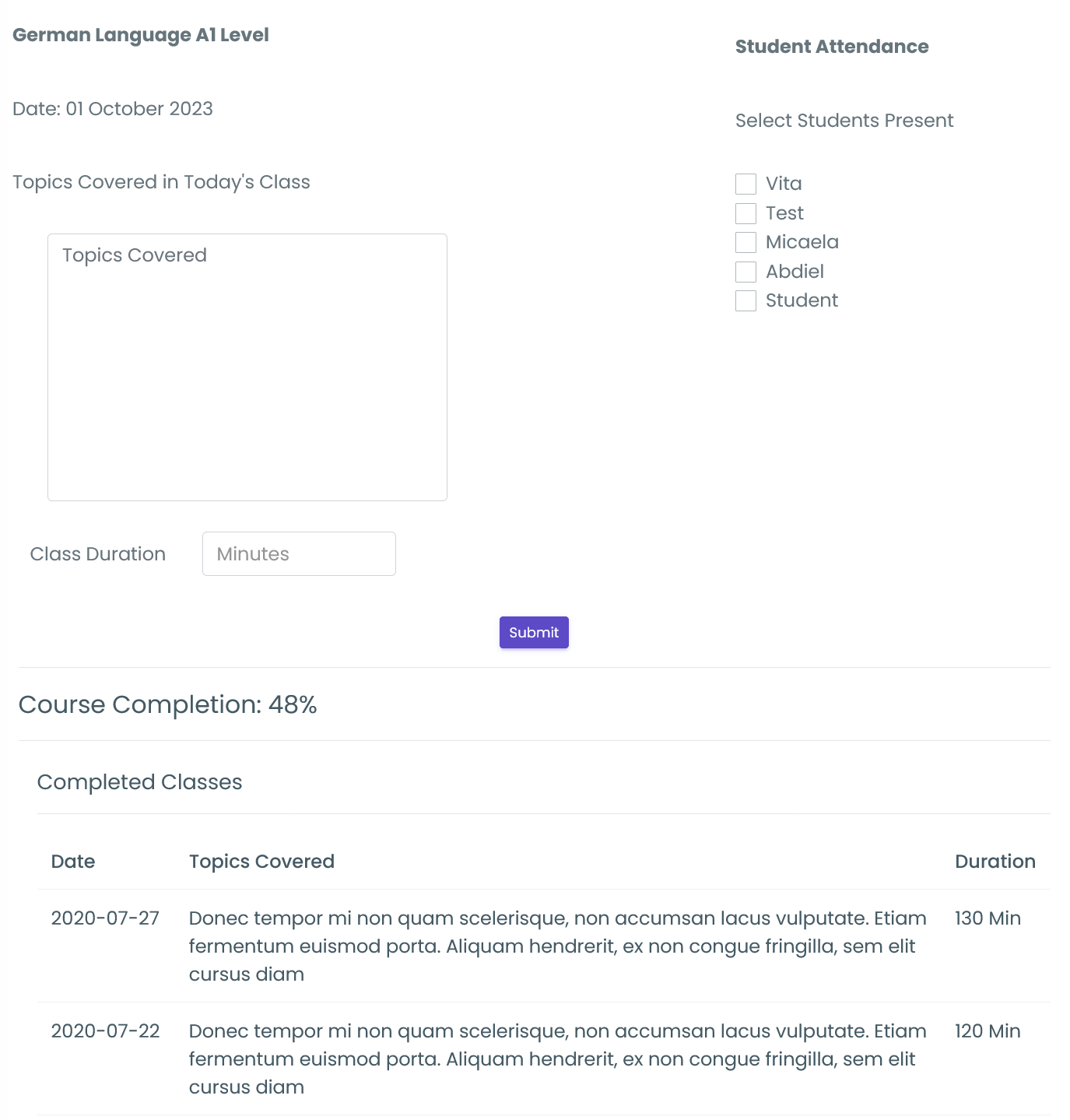This image is a screenshot of a language training course app or website, specifically designed for learning German at the A1 Level. The layout is primarily composed of black text on a white background, formatted in portrait orientation without defined borders.

In the top left corner, there is a bold header stating "German Language A1 Level" followed by the date "01 October 23." Directly below this, there is a section titled "Topics covered in today's class" which currently has a blank space for listing topics.

To the right, another bold header reads "Student Attendance." This section instructs users to select students present and features names with corresponding checkboxes. The listed names are Vita, Test, Mikola, Abdiel, and Student.

Below the attendance section, there is a box labeled "Class Duration," with a field for entering the duration in minutes. Centrally located near the middle of the screen is a prominent purple rectangular button labeled "Submit" in white font.

Further down, a heading titled "Course Completion" indicates a 48% completion rate. A subheader labeled "Completed Classes" displays details in a tabular format with columns for dates, topics covered, and duration. The first entry shows the date "07-27-2020" with a duration of 130 minutes and a description of the covered topics. The second entry lists "07-22-2020," a duration of 120 minutes, and also includes a detailed description of the topics covered.

Overall, the screenshot provides a comprehensive view of a German language course's progress, student attendance, class duration, and topic coverage, all organized neatly for easy reference and updating.